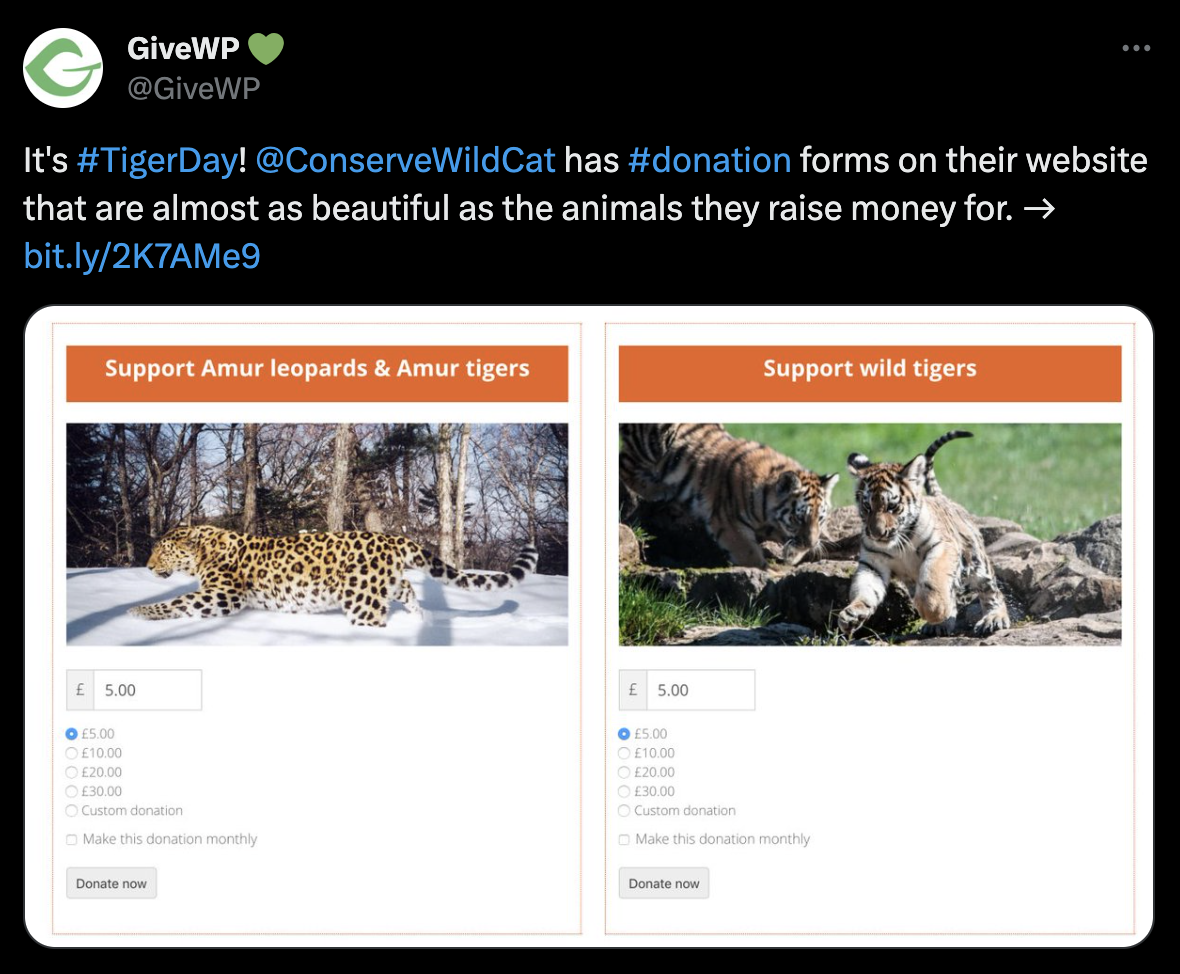This detailed caption could be:

A cropped and enlarged screenshot of a tweet by the user 'givewp' with the handle @givewp. The user profile picture is a stylized leaf oriented sideways to resemble a 'G', complemented by a green heart emoji in the username. The tweet, celebrating #TigerDay, reads: "It's #TigerDay! @ConserveWildcat has #donation forms on their website that are almost as beautiful as the animals they raise money for," followed by a right-pointing arrow leading to a website link.

Attached is a large thumbnail showcasing two parallel donation forms. The left form is dedicated to 'Support Amur Leopards and Amur Tigers,' and the right form is focused on 'Support Wild Tigers.' Each form features a striking photograph of the respective animal above a text box for donation entries, with options for preset donation amounts. The forms are completed with a 'Donate Now' button in grey.